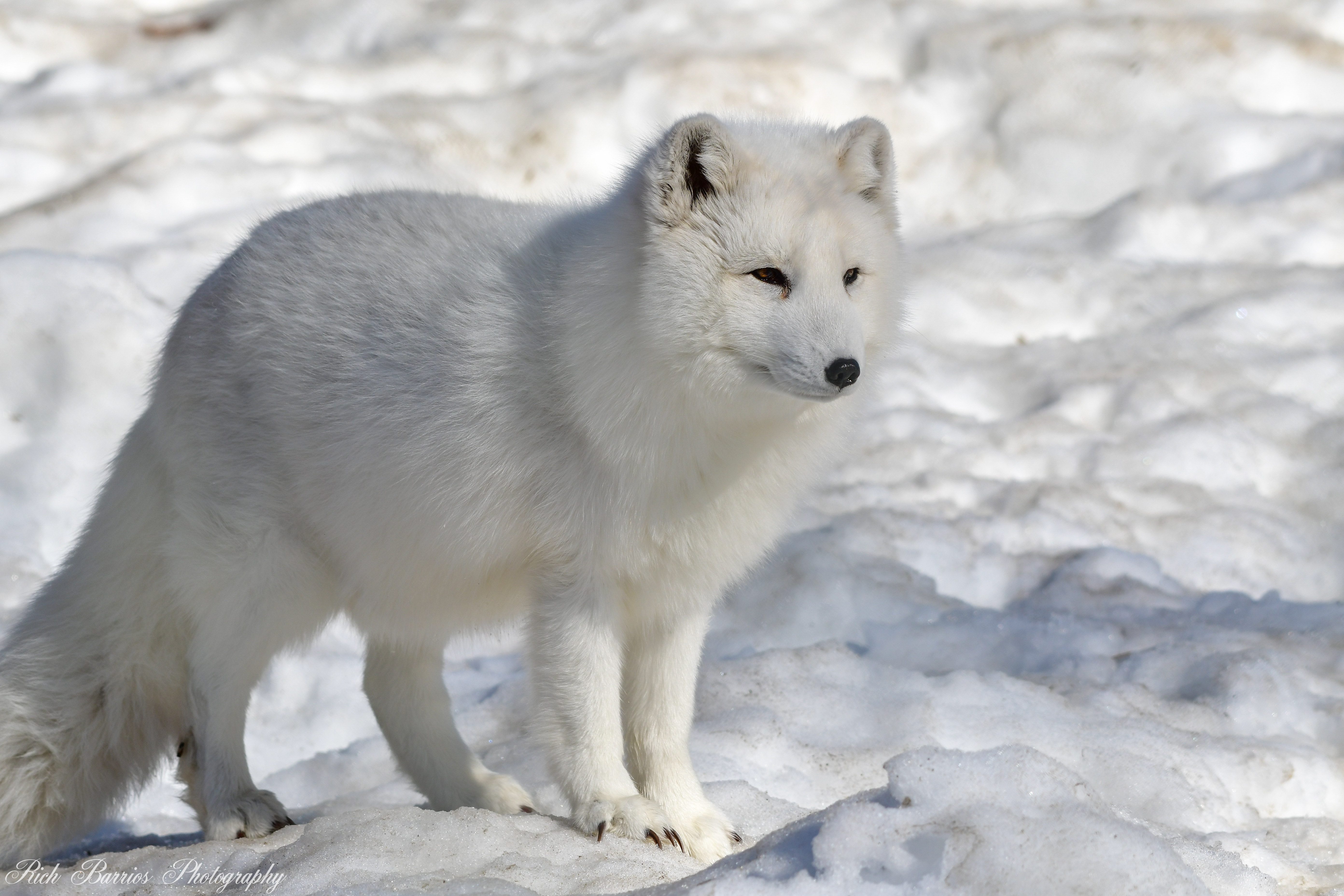The image showcases a pristine arctic scene with an arctic fox poised gracefully in the middle of the frame. The entire background is a textured expanse of snow, resembling puffy clouds with small mounds and gentle hills that extend all the way to the horizon. The midday sun, coming from the right, casts a soft glow over the scene, highlighting the fox and its surroundings. 

The fox has a strikingly white, fluffy coat, a bushy tail, and long, sharp black claws on its furry feet. Its face features a medium-length snout, a black nose, and dark, focused eyes. Its ears are perked up, indicating alertness and readiness for action. The fox is captured looking intently to the right, exuding a sense of determination and focus. 

In the bottom left corner, the photograph is subtly signed "Rich Barrios' photography" in white cursive, lending a professional touch to this realistic and captivating image.